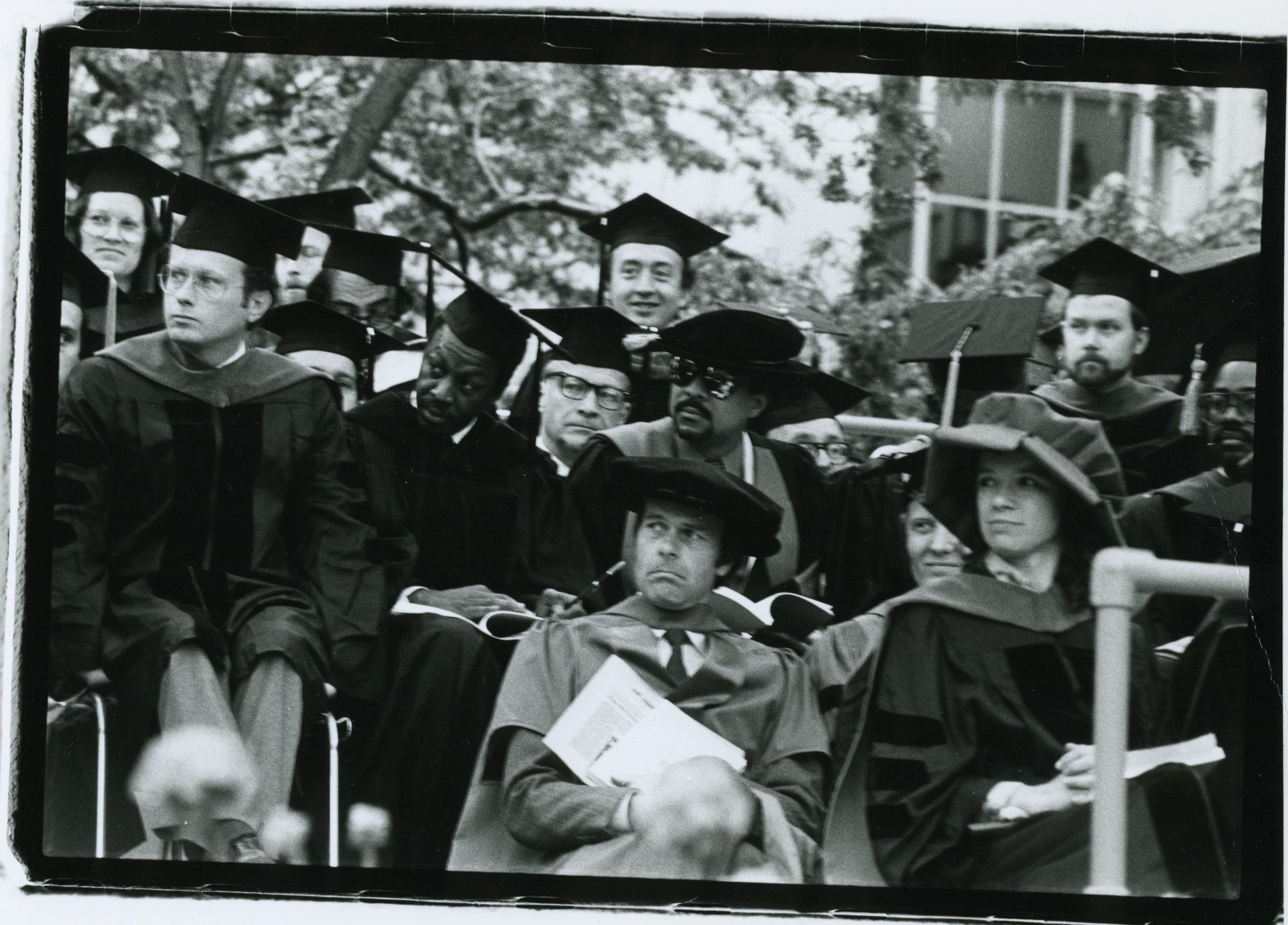In this striking black-and-white photograph, taken outdoors during a graduation ceremony, numerous individuals clad in traditional black caps and gowns are seated on a tiered stage, with a backdrop featuring a building in the top right and tree foliage in the top left. These individuals are mostly professors, positioned in layered rows from bottom to top, predominantly looking towards the left as if captivated by a speaker off-frame. At the forefront, there are two notable individuals: a gentleman in a lighter-colored robe with a stack of papers across his lap and a slight frown, and a woman wearing a distinctive, almost baker's hat and a black robe, with her hands folded in her lap. Among the diverse group, there are several white and African-American figures, some with glasses. The overall scene suggests a moment of focused attention and solemnity, emblematic of the gravity and anticipation typical of a graduation ceremony.